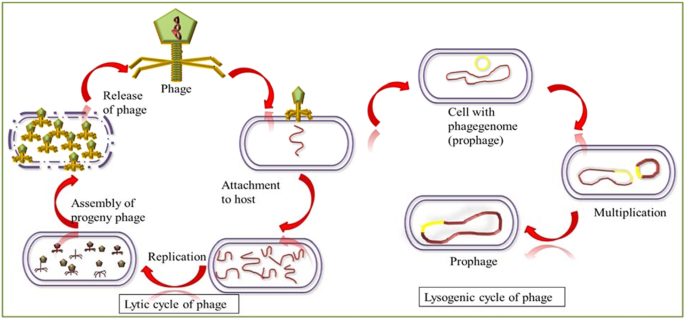This image on a white background with a thin light green border features detailed educational slides illustrating the lytic and lysogenic cycles of bacteriophage infection in a flowchart-like format. The page is divided into two main sections. The left section depicts the lytic cycle of phage, starting from a green pentagon at the top labeled "phage," followed by red arrows leading sequentially to boxes titled "attachment to host," "replication," and "assembly of progeny phage," and ending with "release of phage." Each box contains simple drawings, including a spiral shape representing DNA and pentagon-shaped structures depicting bacteriophages at various stages.

The right section illustrates the lysogenic cycle of phage. It begins with a red arrow that transitions from "attachment to host" through several stages, including a labeled box "cell with phage genome (prophage)," "multiplication," and then "prophage." Each stage is represented by simple drawings, such as a spiral and split structures illustrating the phage genome's integration and replication within the host cell. 

Throughout both cycles, red arrows connecting these labeled stages depict the progression of events. At the bottom of each section, the labels "lytic cycle of phage" and "lysogenic cycle of phage" clearly indicate the respective processes being described. The diagrams offer a vivid visual explanation of how bacteriophages interact with their host cells, providing a clear comparison of the two infection cycles.